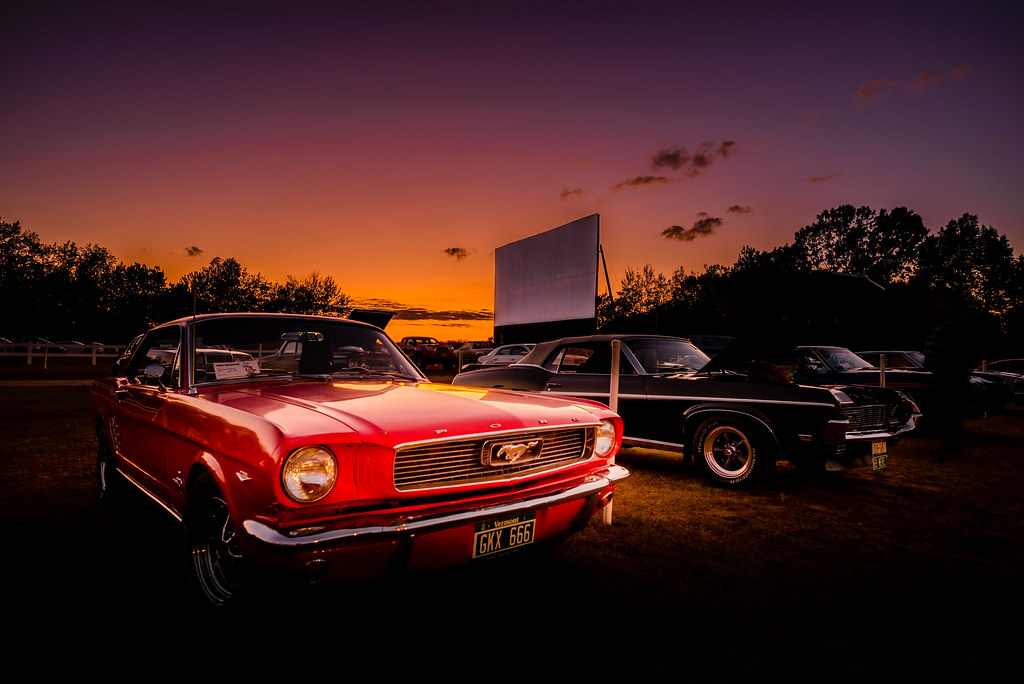In this captivating image of a drive-in theater at sunset, a stunning red, older model Ford Mustang with the license plate GKX666 takes center stage. The Mustang, gleaming in the fading light, is parked facing slightly to the right, away from the giant theater screen that looms in the background. Next to it, a classic black muscle car with shiny gold rims adds to the nostalgic atmosphere. Several other vehicles are scattered throughout the lot, basking in the mixture of dark purple, lavender, and bright orange hues of the sky. The scene is set with trees surrounding the theater, harking back to a bygone era where cars and outdoor movie experiences ruled the night.